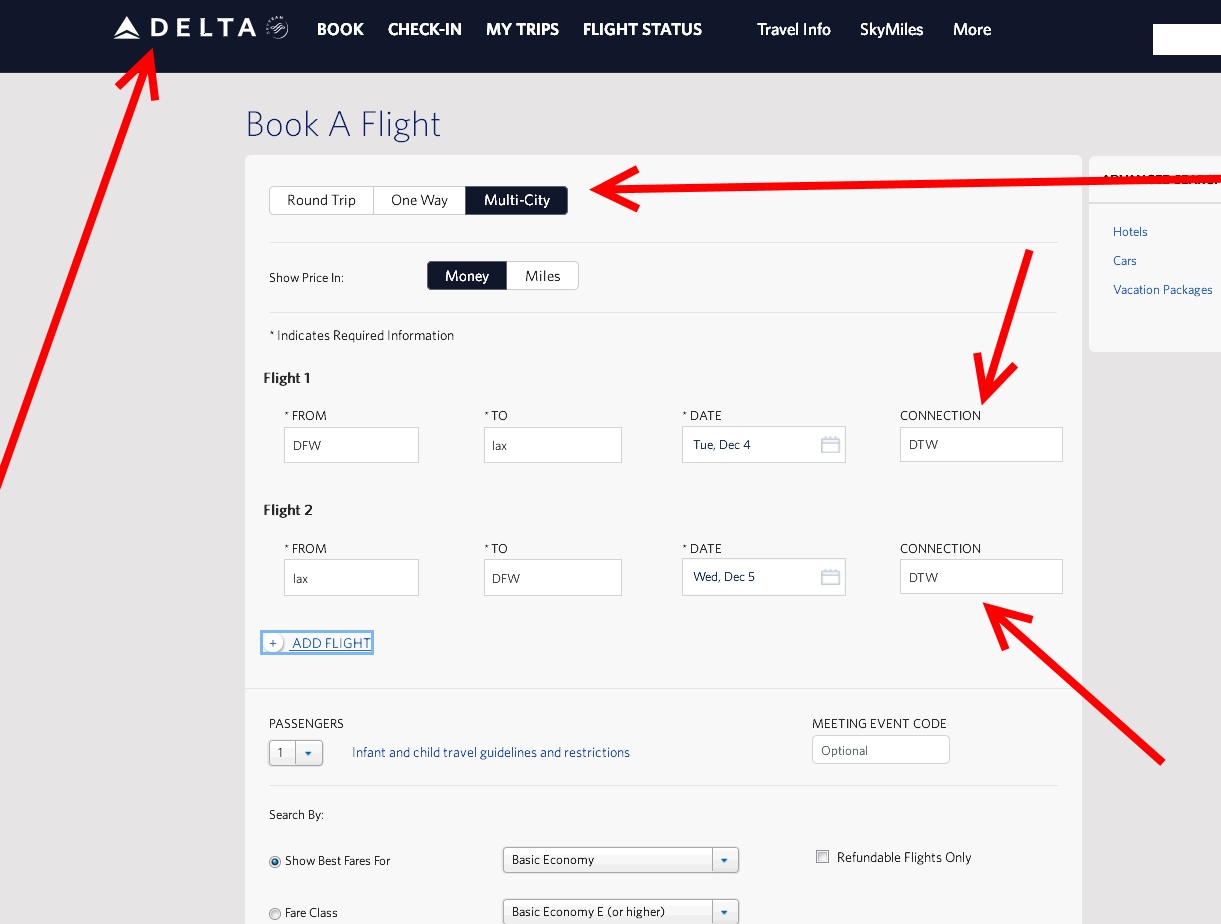This detailed screenshot captures a webpage from Delta Airlines, specifically designed for booking flights. At the top of the page, a sleek black banner features the word "Delta" alongside the airline's iconic logo, all in contrasting white letters. To the right of the logo, the banner includes several navigation buttons in white text for easy access to different sections: "Book," "Check-in," "My Trips," "Flight Status," and "Travel Info."

Directly below the banner, the booking section of the webpage unfolds against a muted gray background. This section is user-friendly and allows input for various necessary details to book a flight. The fields include options to specify your departure ("From") and destination ("To") locations, select travel dates, add additional flights, and choose the number of passengers. There are also options to navigate to booking hotel stays and rental cars, integrating all travel needs conveniently.

Adding a layer of interactive guidance, several red arrows are visible on the screenshot. These arrows likely serve as a training tool, directing the user's attention to key areas of the booking process.